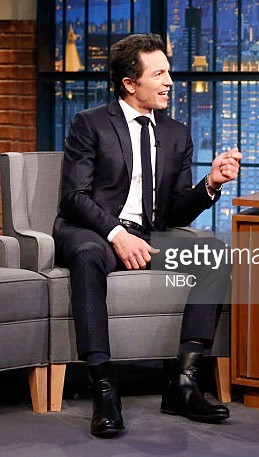The image depicts a modern talk show set that closely resembles the Tonight Show. In the foreground, a man is seated comfortably in a gray cushioned chair with thin armrests and wooden legs. He is dressed in a gray suit with a matching thin tie, a white button-down shirt, a black belt, black socks, and black shoes. His brown hair is visible, and his mouth is open mid-conversation. His left hand is gesturing, bent at the elbow, while his right arm rests on his lap. Another identical gray chair is positioned to his left. The floor is covered in gray carpeting. In the background, a red brick wall is visible on the left, and there's a window showing a cityscape with the lights of the buildings against a blue backdrop, suggesting it is a fake city view. To the right, part of a desk is seen, indicating where the talk show host would sit. Toward the lower middle-right, a watermark reads "Getty Image," with part of the text cut off, and "NBC" underneath it in white text.